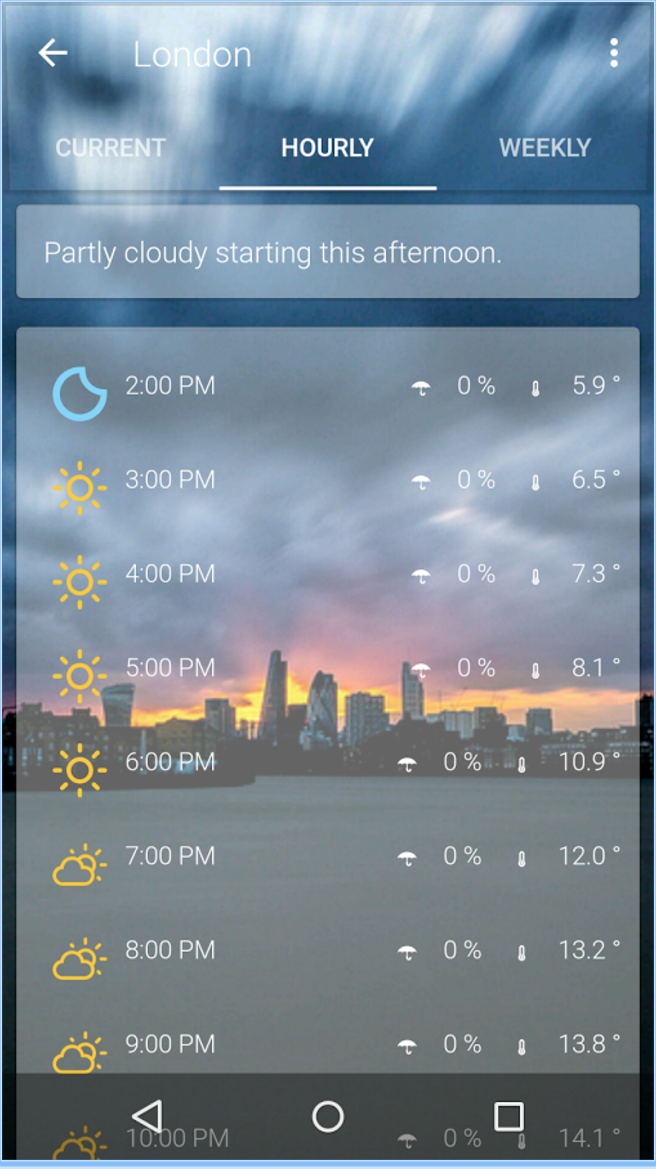This screen capture displays a detailed hourly weather forecast from a weather app for the location of London. The backdrop features a scenic image of London during what appears to be either sunrise or sunset on a rather cloudy day. The information overlay is structured in a clean, easy-to-read column format.

On the left column, the current time slots range from 2 PM to 9 PM. Each row includes a weather icon indicating the conditions for that hour, followed by the percentage chance of precipitation, and the temperature in degrees Celsius:

- **2 PM:** Partly cloudy, 0% chance of precipitation, 5.9°C
- **3 PM:** Sunny, 0% chance of precipitation, 6.5°C

This pattern continues hourly, showing a consistent 0% chance of precipitation, with temperatures gradually increasing up to 13.8°C by 9 PM.

At the top of the screen, the 'Hourly' tab is highlighted, distinguishing it from the 'Current' and 'Weekly' options in the app's ribbon. Below the tabs, a brief summary states, "Partly cloudy starting this afternoon."

Though the exact date is not provided, this screen capture effectively showcases an hour-by-hour breakdown of London's weather conditions, emphasizing clear skies and a warming trend into the evening.